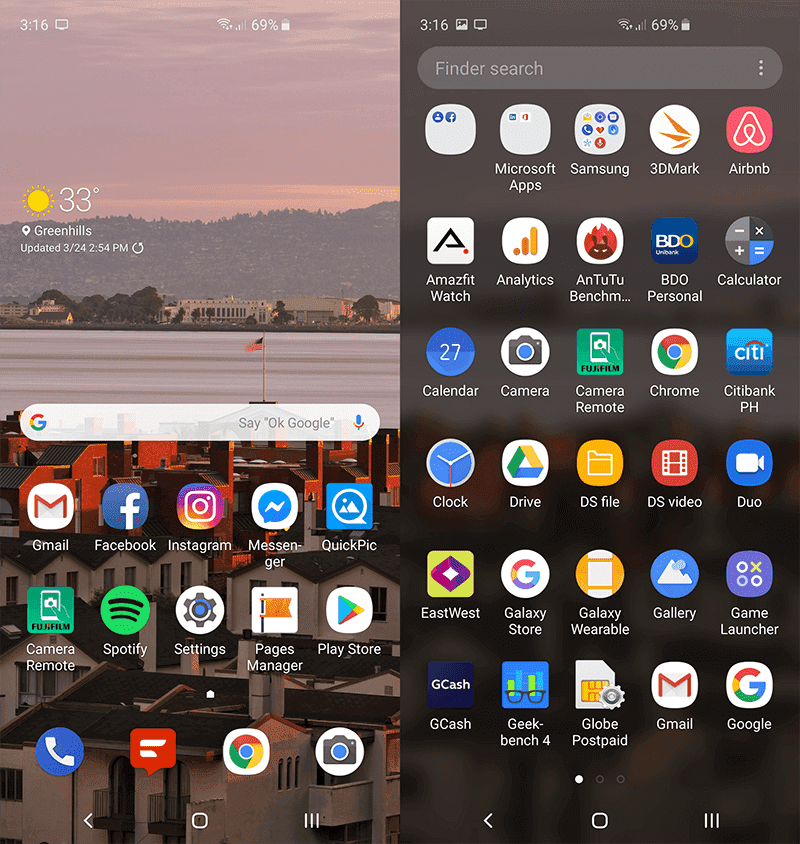This image appears to be a screenshot of an Android device, likely a Samsung tablet. At the top left corner of the screen, the status bar displays the time as 3:16, with a full Wi-Fi signal, a cellular signal strength of 2 out of 4 bars, and a battery level at 69%. An icon indicating sunny weather with a temperature of 33 degrees Celsius is also visible. The location is specified as Greenhills, with the weather information last updated on March 24th at 2:54 p.m., accompanied by a refresh button.

The font predominantly used in the screenshot is white. The background image seems to feature a picturesque scene that includes a body of water, some industrial buildings, lush forestry to the left, and a larger metropolis further in the background. In the middle of the body of water, an American flag on a flagpole is visible, waving in the wind.

Directly below the scene is the Google search bar, designed as a white pill-shaped button that prompts the user with "Say OK Google" and includes a microphone icon to its right. The home screen also displays several app icons, including Gmail, Facebook, Instagram, Messenger, and QuickPic.